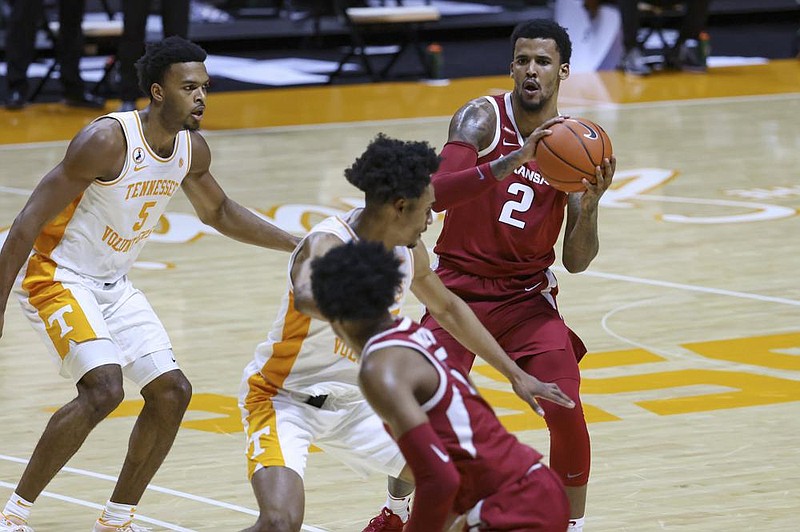In this photograph of a high-intensity basketball game, there are four players centrally positioned on a pale wooden court, engaged in a spirited play. Two players wear the white uniforms of the Tennessee Volunteers, accentuated with burnt orange details, which make the Tennessee team affiliation clearly visible. The opposing team, dressed in maroon or wine-colored uniforms with white striping and numbering, is likely Arkansas.

The central focus of the image is a player in maroon, positioned towards the right side of the photograph. He holds the basketball in front of his left shoulder, leaning slightly to the right, appearing to strategize his next move. His concentrated gaze suggests he is in the midst of communicating or preparing a pass. Flanking him, two Tennessee players in white and orange are actively defending, bent at the knees and ready to move.

A fourth player, dressed in maroon, has his back to the camera, also in a crouched position, watching the interaction between his teammate and the defenders. The background reveals a section of the court with distinctive white and orange markings along the sidelines, indicating it's a home game for Tennessee. Above the scene, a glimpse of a black area, possibly a bench or mat, and a few individuals in black pants are visible, adding to the bustling ambiance of the game. All the players depicted are African-American, sporting short, neat hairstyles. The image captures a moment brimming with energy and focus, characteristic of a competitive basketball match.